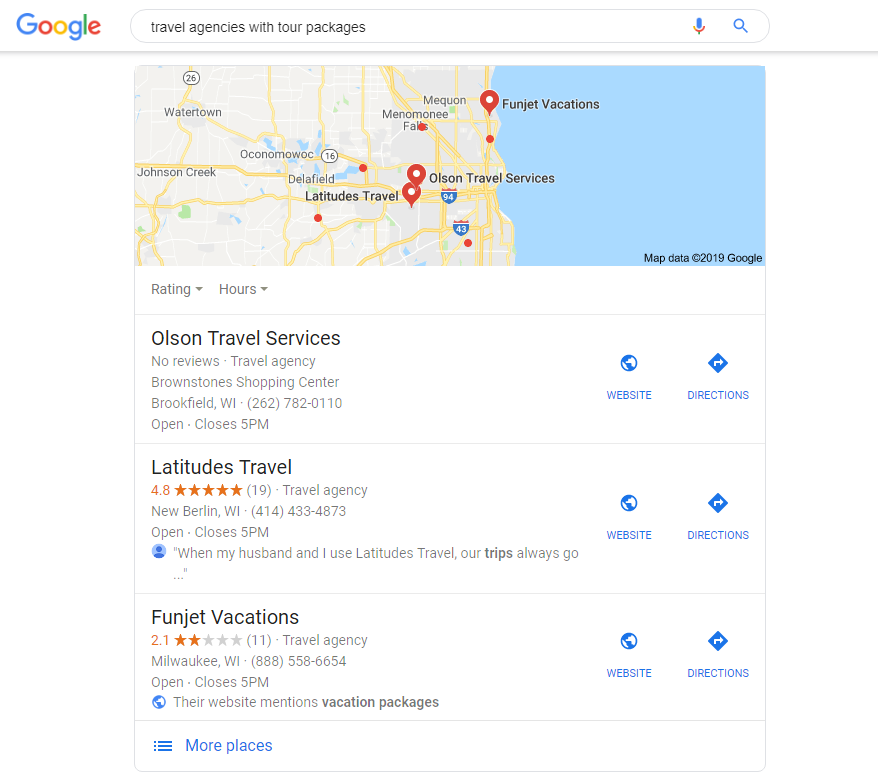A screenshot of a Google search results page highlights travel agencies with tour packages. In the top left corner, the colorful Google logo is prominently displayed, featuring a capital "G" in blue, followed by lowercase letters: "o" in red, "o" in yellow, "g" in blue, "l" in green, and "e" in red. Below the logo, a long white search bar stretches across the screen with the query "travel agencies with tour packages" typed inside it. To the right end of the search bar sit a blue microphone icon and a blue magnifying glass icon, signifying voice search and search functionalities, respectively.

Beneath the search bar is a detailed map showing the area around Watertown and Johnson Creek, bordered by an ocean. The map is marked with multiple red pins indicating the locations of various travel agencies. Yellow gridlines denote the roads, while blue interstate signs with red tips represent major highways, including Interstates 94 and 43.

At the bottom of the map are details for several travel agencies. The Olson Travel Agency is listed first, providing comprehensive information including reviews, its address, and operating hours. To the right are buttons for the website and directions. Below Olson Travel Agency are two more listings: Latitudes Travel, which boasts a 4.8-star rating with accessible reviews, and Fun Jet Vacations, which has a 2.1-star rating based on 11 reviews.